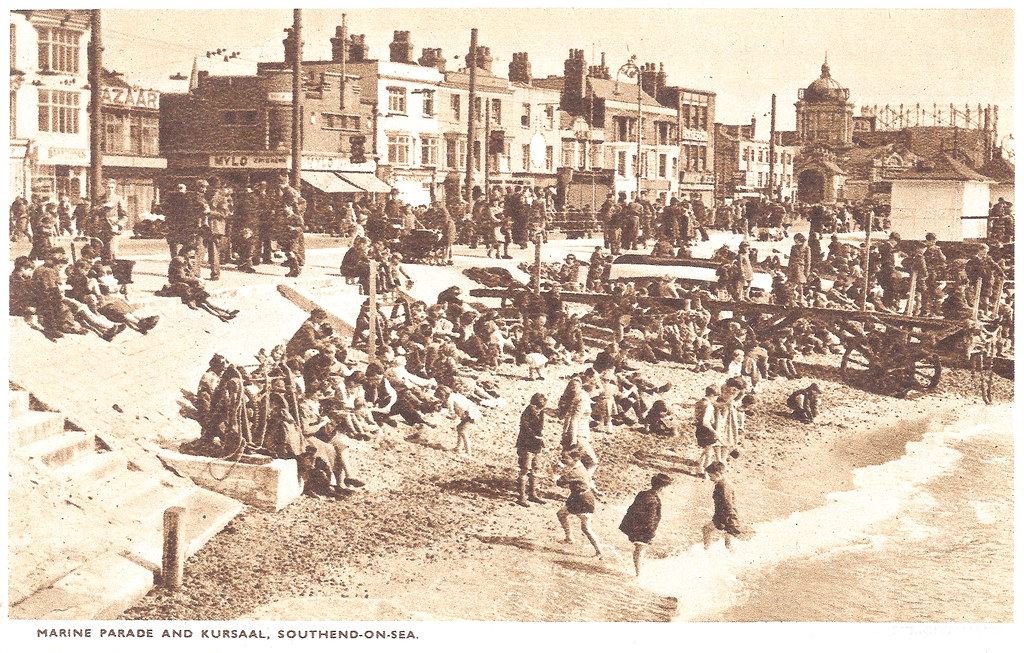A sepia-toned vintage photograph, possibly from the turn of the century, depicts a bustling beach scene with a cityscape in the background. The image is labeled at the bottom with the words "Marine Parade and Kursaal, Southend-on-Sea". The photograph captures throngs of people, predominantly clothed in formal wear, scattered throughout the scene. Children can be seen playing at the water's edge, where the waves meet the sandy shore. Central to the image is a long wooden board with metal wheels, likely part of a large wagon or flatbed, possibly used for launching boats.

The beach is lined with steps on the left-hand side, leading up to a crowded urban area filled with three-story brick buildings, some adorned with chimneys and awnings. Notable signage includes "Bazaar" and "Milo" on the storefronts. The street is equipped with high-arching lampposts illuminating the area. A group of men appears to be carrying an inverted canoe or rowboat in the background, hinting at nautical activities. The overall composition presents a lively seaside town, filled with individuals of all ages and possibly hosting a parade or public gathering, reflective of its historical charm and the community's vibrant spirit.